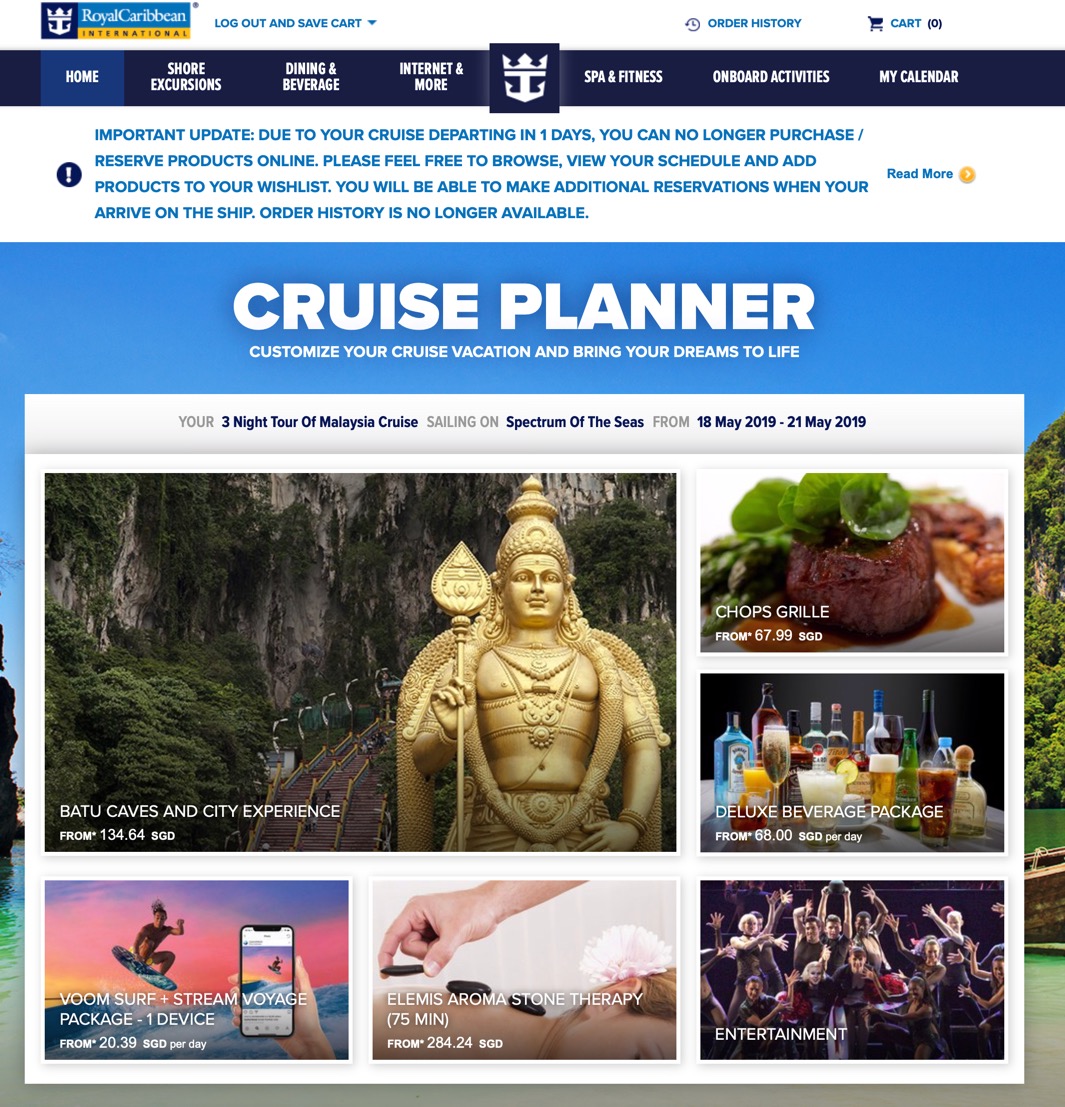This detailed screenshot captures the homepage of the Royal Caribbean International Cruise Site. In the upper left corner, the Royal Caribbean logo is prominently displayed with an anchor and crown badge, alongside the text "Royal Caribbean" on a lighter blue field, and "International" underlined in gold. 

To the right, options such as "Log out," "Save Cart," and "Order History" are provided, along with an empty cart icon at the far right. The main navigation menu includes "Home," "Shore Excursions," "Dining & Beverage," "Internet & More," "Spa & Fitness," "Onboard Activities," and "My Calendar," with "Home" highlighted in a lighter shade of blue.

An important update message appears beneath the main menu, alerting users that, due to their cruise departing in one day, they can no longer purchase or reserve products online but can still browse, schedule, and add items to their wish list. Additional reservations can be made onboard.

The page is titled "Cruise Planner," with the text appearing boldly across a photograph that suggests an exotic destination, possibly Thailand. Below this, the tagline "Customize your cruise vacation and bring your dreams to life" is displayed, inviting users to personalize their experience.

A panel of tiled photos invites further exploration. The largest tile in the upper left highlights the "Batu Caves and City Experience," featuring an image of a golden idol. Below it, the "Voom Surf & Stream Voyage Package" is represented. To the right, "Chop's Grill" showcases a sumptuous steak, and beneath it, the "Deluxe Beverage Package" is pictured with a variety of alcoholic drinks. In the bottom row, an "Entertainment" section features individuals at a sporting event, while the "Elemis Aroma Stone Therapy" shows hot stones being placed on a person's spine during a spa treatment.